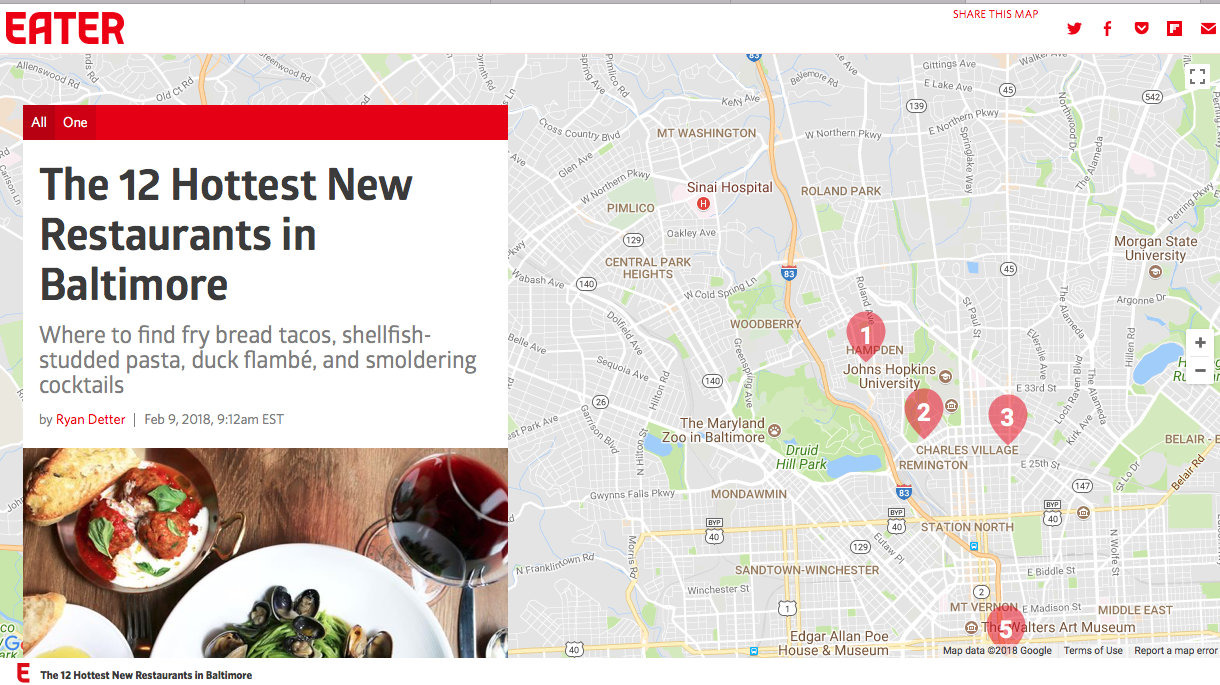At the top of the page, the word "EATER" stands out prominently in bold red letters. Below it, a gray rectangular map is displayed, highlighting the Maryland Zoo in Baltimore, indicating that this is a map of Maryland. 

On the left side, there is a red rectangle with the words "ALL" and "ONE" in white letters inside it. Directly beneath this, bold black letters announce "The 12 Hardest New Restaurants in Baltimore." Following this headline, a short paragraph details where one can find fried bread tacos, shellfish-studded pasta, duck flambé, and smoldering cocktails.

At the center-right of the page is a photo featuring a glass of red wine accompanied by plates of food. One plate holds bread and what appears to be meatballs, while another plate showcases shellfish garnished with greenery. 

In the bottom left corner, another plate is visible displaying bread alongside an unidentified creamy light brown substance. The map on the right side of the page is marked with red teardrops numbered 1, 2, 3, and 5, although number 4 is noticeably absent.